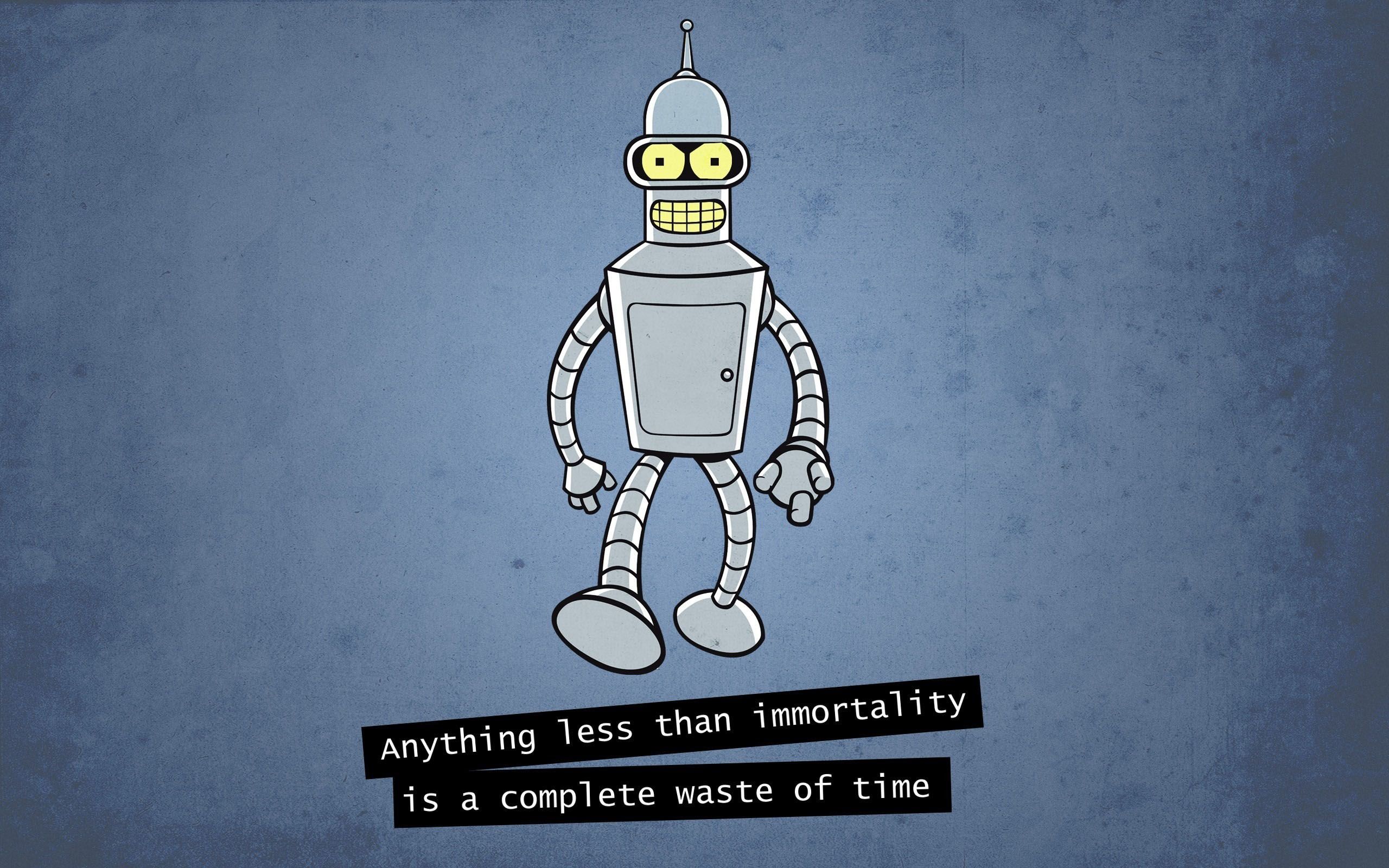This detailed sketch captures Bender, the iconic robot character from the animated television series "Futurama," in mid-stride. Bender is depicted in a walking motion, with his metallic arms hanging loosely by his sides and his segmented legs in motion. His mouth is wide open, and his characteristic big, round yellow eyes add to his expressive look, highlighted by the small antenna perched atop his head. The robot's body features his signature small chest door and the segmented design of his limbs emphasizes his mechanical nature. The background consists of a blue field with black patches, creating a textured look that mimics a real wall. At the bottom of the image, two black boxes contain text. The first line of text, slightly tilted, reads, "Anything less than immortality," while the second, horizontally aligned, completes the thought with, "is a complete waste of time." This thorough depiction brings Bender's quirky personality and existential musings to life.